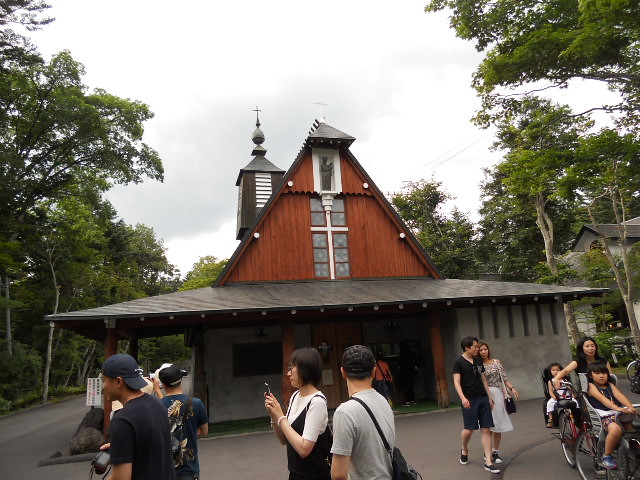This outdoor daytime photograph captures a small temple or church surrounded by trees and pathways. The building features cement outer walls, a metal arching roof, and a wooden triangular top with a small steeple. At the top of the building, a statue is embedded in a recessed area that appears like a window but serves as a display niche. The sky above is largely overcast with only patches of blue visible through the white clouds.

In the ambiance of a probable park area, various people are depicted walking across the cement or asphalt surface in the foreground. A couple is seen in the center; the man gazes towards the temple while the woman looks at her phone. In the bottom right corner, there are children in wheelchairs and a couple walking away. Additionally, two men are seen in the distance heading away from the temple, which someone else is entering, though they are not clearly visible. The overall scene suggests a tranquil public space frequented by families and individuals alike.